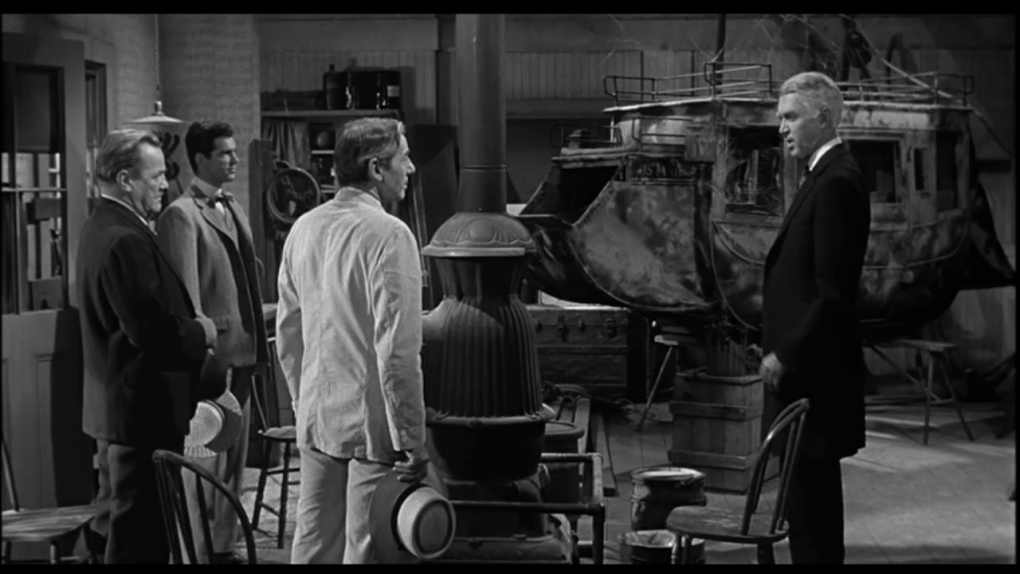This detailed black-and-white still from an old movie features four men dressed in period-appropriate business suits, arranged around a central pot-bellied stove typical of the early to mid-1800s. The scene includes three men on the left, with one man in a light-colored suit holding a hat by his side, and another in a gray suit, while the third man stands in a dark suit. Facing them on the right is a distinguished, taller man in a black suit, likely portrayed by James Stewart, who appears as an elderly gentleman with white hair.

In the background behind Stewart, a stagecoach, conspicuously propped up on sawhorses without its wheels, suggests a setting in a repair shop or storage area, characteristic of Western times. Surrounding the stove and the men are several antique items, including old wooden buckets, crates, and an old set of doors with a pull-down shade. The room's unique composition creates a vivid, dynamic snapshot, highlighting the intricacies of the period and the tense interaction between the characters.